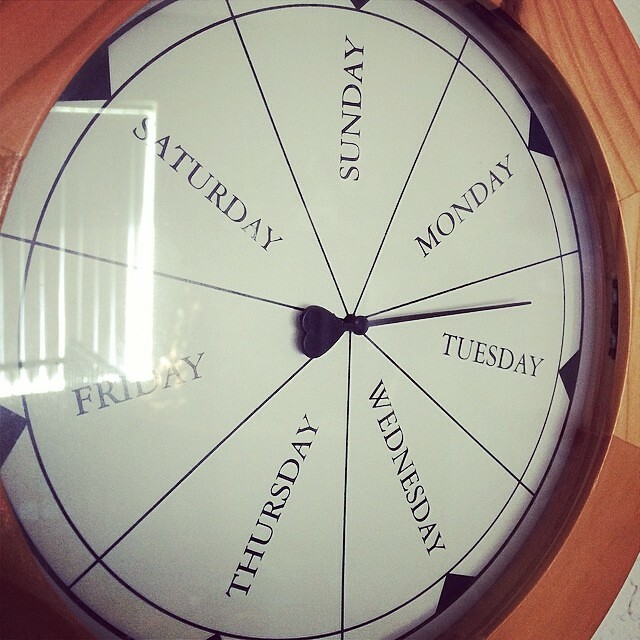The image showcases a unique wooden device resembling a clock, but instead of traditional numbers, the circular face displays the days of the week, arranged like pizza slices. Each "slice" marks a different day, starting with Sunday at the top and ending with Saturday. The clock features a central hand with a heart at its base and a rounded tip at the other end, pointing to the current day. This hand might spin, indicating anything from daily schedules to themed nights like date nights or Netflix marathons. The white clock face is bordered by dark wood and is mounted on a larger, lighter wooden base. There are reflections visible on the clock's glass surface, with a fence appearing over the Friday and Saturday sections and blinds faintly visible in the background.